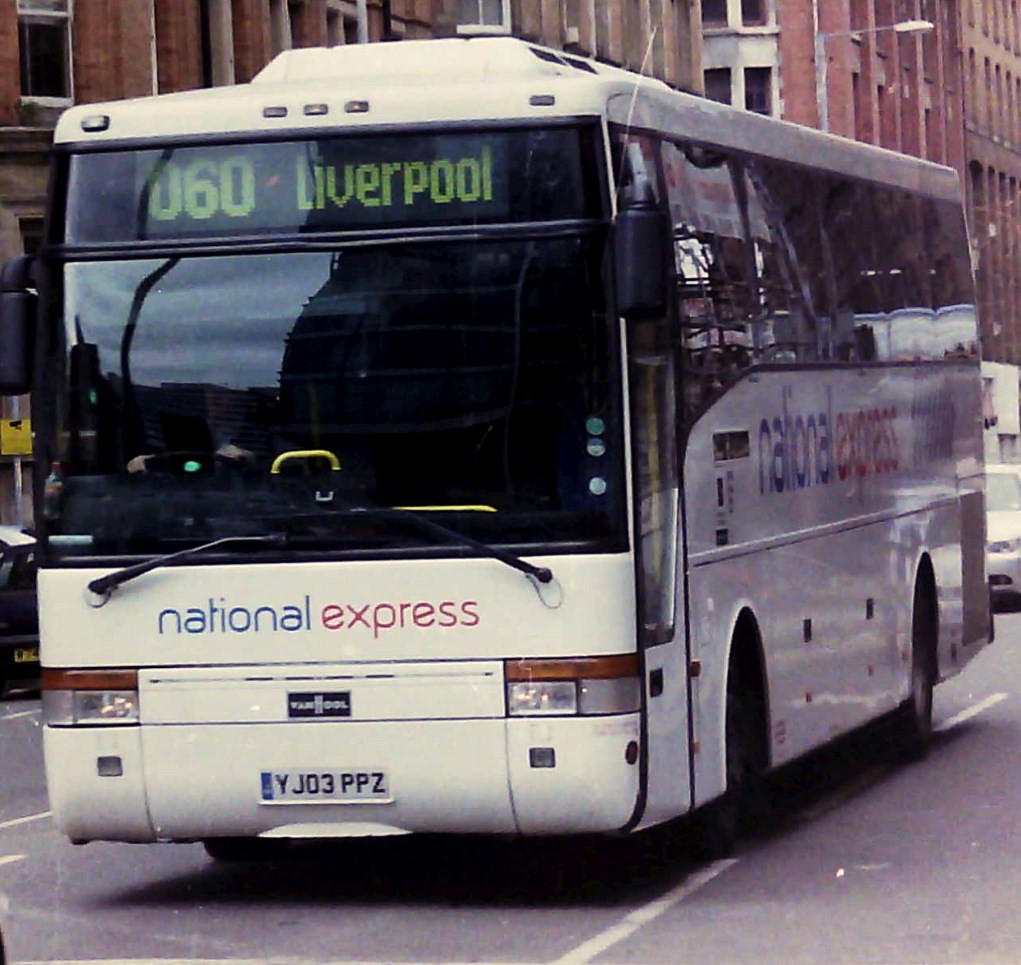The image captures a white public bus, prominently displaying "National Express" in blue and red letters below its windshield and along its sides. On the digital sign above the windshield, it reads "060 Liverpool." The bus features a flat-front design and European license plate "YJ03PPZ." Behind the bus, a white car follows, and both vehicles are seen on a street lined with markings and street lights. Reflections of nearby structures are visible on the bus windows and windshield, indicating the scene is set amidst tall, red-brick buildings with numerous windows. The photo, taken during the daytime under natural light, highlights the urban environment in which the bus is traveling.